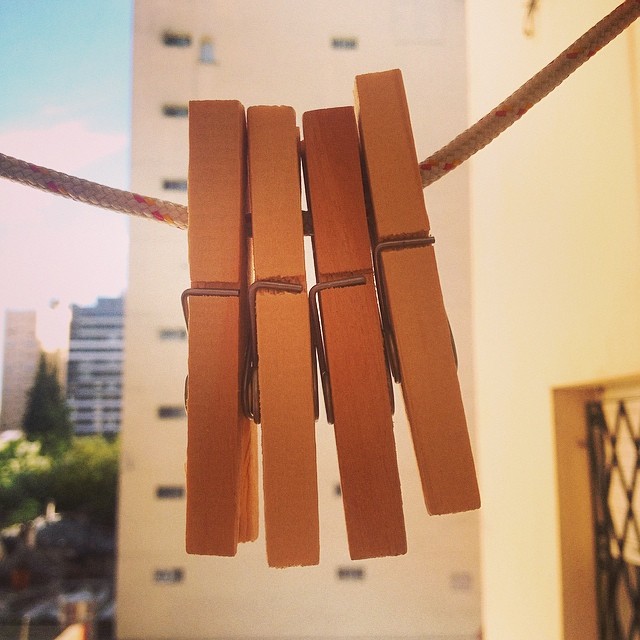This extreme close-up photograph captures four wooden clothespins, varying in light and dark brown hues, securely fastened to a weathered white clothesline, now spotted with small pink and yellow dots, as well as red and black stains. The clothespins are held together by metal springs that curl at the edges to create tension. To the right, there is a grated window with a diamond-patterned black metal mesh, which contrasts sharply with the blurred, yet discernible backdrop of tall city buildings. These buildings, displaying a range of cream, tan, gray, and black, rise behind a line of foliage that includes dark and light green trees. The photograph, taken during the day under an overcast sky filled with white clouds and patches of blue, illustrates the juxtaposition between the intricate details of the foreground elements and the expansive urban scene in the background.